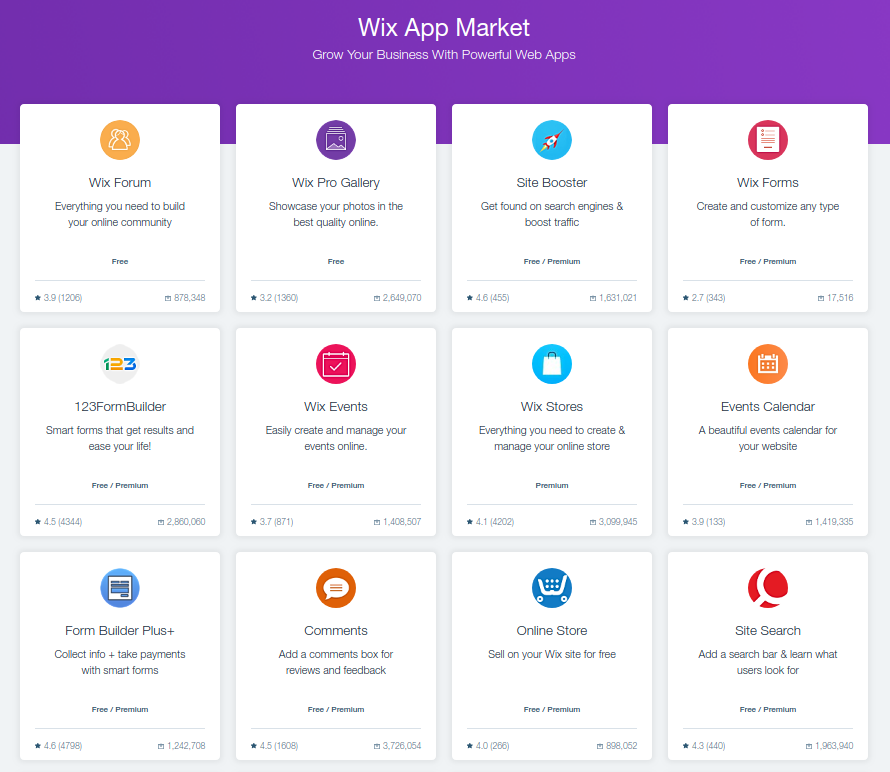The image showcases a section of a Wix website, specifically highlighting the Wix App Market. Set against a rich purple background, the top portion of the page prominently features the header "Wix App Market" accompanied by a subtitle, "Grow Your Business with Powerful Web Apps." Below this, the screen is arranged into a grid of 12 square tiles, each representing a different Wix app available for use. 

These apps include:
1. **Wix Forum**
2. **Wix Pro Gallery**
3. **Site Booster** (icon: a rocket in the sky)
4. **Wix Forms**
5. **123 Form Builder**
6. **Wix Events**
7. **Wix Stores**
8. **Events Calendar** (icon: a calendar)
9. **Form Builder Plus**
10. **Comments** (icon: a speech bubble with text)
11. **Online Store**
12. **Sites**

Each app tile features a unique, colorful icon that makes it easily recognizable, as well as a brief one-liner description underneath. The tiles also display ratings and visit statistics at the bottom right corner, providing users with insights into each app's popularity and usefulness. The layout is clean and organized, making it simple for users to explore and choose the apps best suited to enhance their websites.